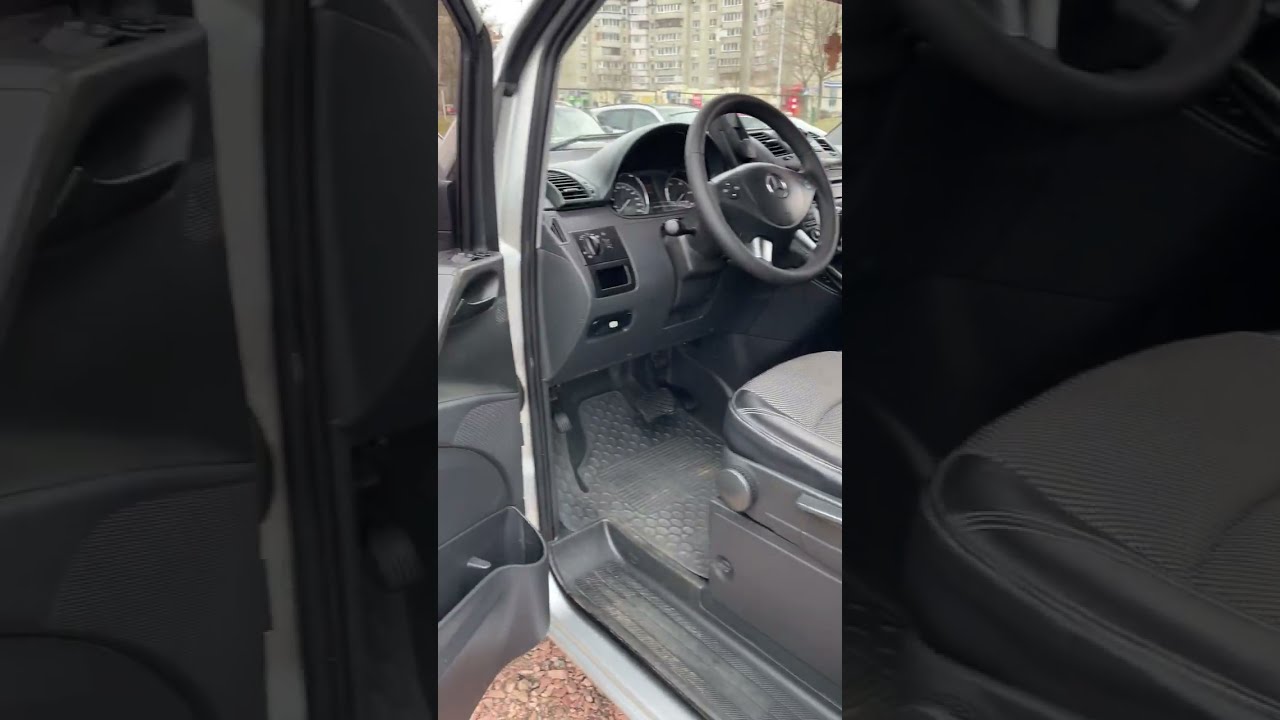The image is divided into three vertical sections, with the first and third sections featuring darkened close-ups of the central section. The central section reveals a detailed photograph of a car's interior taken from outside with an open driver's side door. The car's interior is predominantly gray, featuring a gray leather-like material and a black dashboard. The steering wheel, adorned with various buttons, is clearly visible, as are the gray floor mats and the levers for adjusting the seat.

Additionally, the interior view includes the foot pedals, part of the driver's seat, and the door's runner, which appears slightly dirty. The partially open door exposes the door handle, window, and a small compartment. Through the car's front windshield, multi-story brown apartment buildings and other vehicles on the road can be seen. There are also trees sans leaves and a reddish gravel-like area, possibly a parking lot, visible outside.